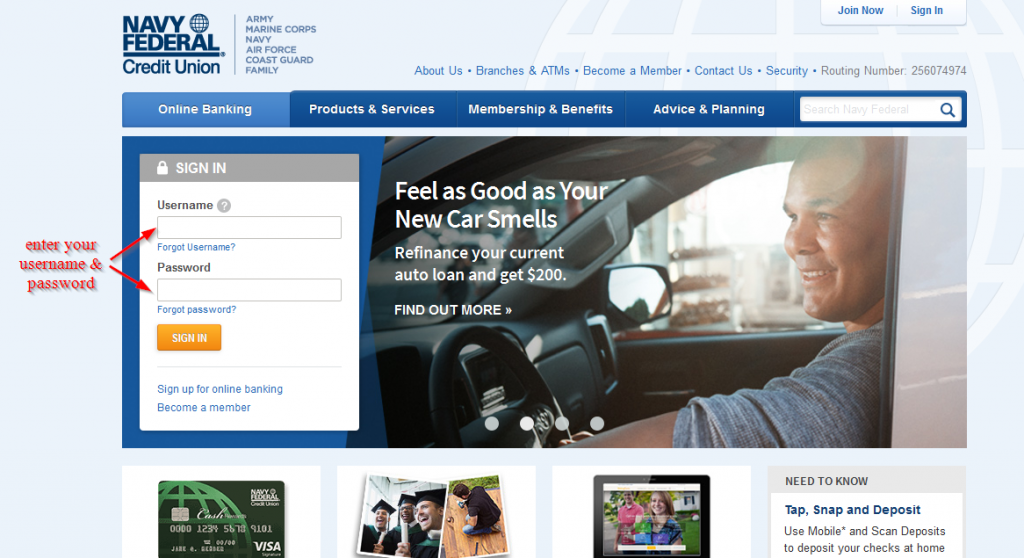The image is a detailed screenshot of a web page from the Navy Federal Credit Union, displayed on a computer screen. At the center of the page, there's a large, visually appealing banner featuring a person within a car, alongside the enticing message: "Feel as good as your new car smells." Directly below this, a subheading reads, "Refinance your current auto loan and get $200," followed by a prompt to "Find out more."

The page layout includes two main navigation menus positioned at the top. The more prominent menu highlights "Online Banking" and offers additional options for "Products and Services," "Membership and Benefits," and "Advice and Planning." 

On the left side of the main image, there is a titled section labeled "Sign In." It features two input fields, one for the username and another for the password, accompanied by an orange "Sign In" button.

Overlaying this webpage screenshot is a tutorial guide, created using red annotations. Two red arrows are prominently pointing to the username and password fields respectively. Adjacent to these arrows is a clear instruction in red text: "Enter your username and password." This superimposed guide is designed to provide a straightforward, foolproof step-by-step process for users, ensuring they know exactly where to input their login credentials.